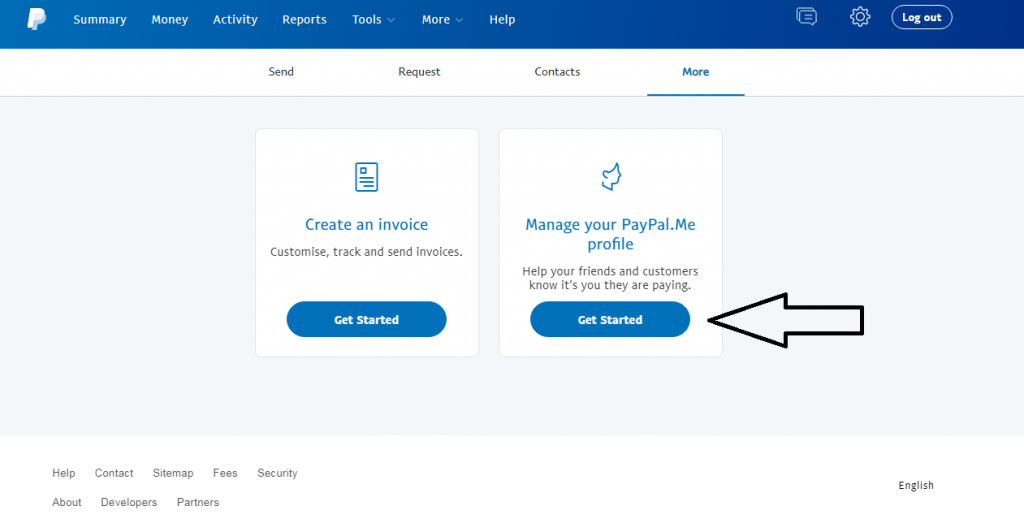The image is a detailed screenshot of the PayPal website interface, highlighting two primary tasks users can perform. 

The upper section of the webpage displays the PayPal logo followed by a navigation bar with clickable options, including "Home," "Summary," "Money," "Activity," "Reports," "Tools," and "More," each with downward arrows indicating drop-down menus for additional choices. To the far right, there are three user icons: one resembling a chat/message function, another for tools, and the third provides the option to log out.

Centrally, the main interface features two prominent square boxes. The first box is dedicated to creating invoices, with the text: "Create an invoice: Customize, track, and send invoices," accompanied by a "Get Started" button for initiating the process. The second box addresses managing a PayPal.Me profile, encouraging users to, "Help your friends and customers know it's you they are paying," also featuring a "Get Started" button.

An additional visual element in the form of a large black arrow points towards these boxes, emphasizing this area as the next actionable step for users. Below this, the interface displays four more options— "Send," "Request," "Contacts," and "More," with the "More" option selected, showcasing the invoice and PayPal.Me management features described above. This provides users with a clear and concise guide to navigate and utilize essential PayPal functionalities.